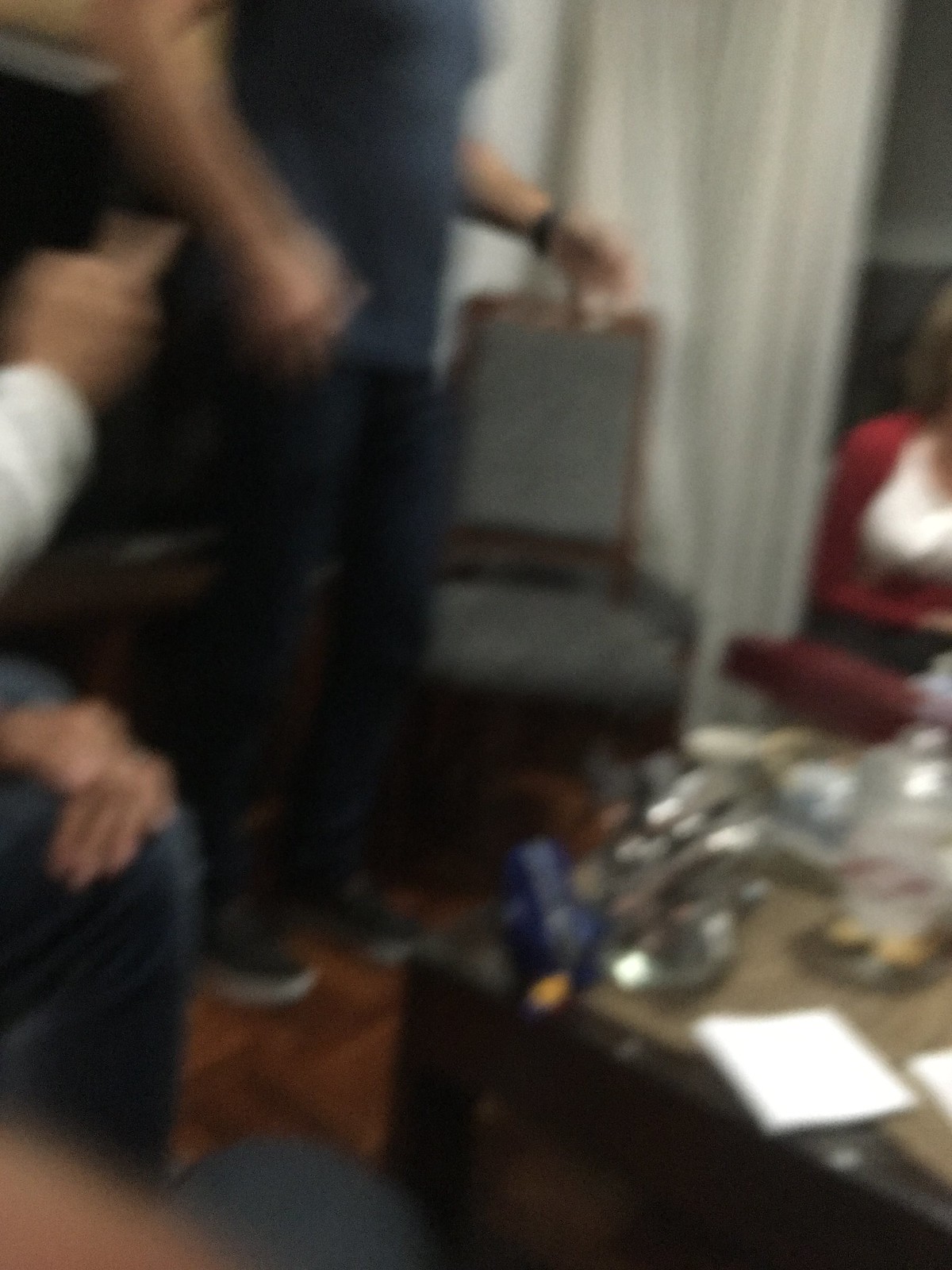This photograph, though somewhat blurry, captures an interior scene within a home. The focal point in the lower right-hand corner is the surface of a coffee table, made from dark brown wood with a tan top. The table is adorned with various glass items, blue objects, and a scattering of white napkins. On the left side of the image, a person's legs, hand, and forearm are visible, extending outward in a white long-sleeve shirt. In the background, in the upper left-hand corner, stands a man in a dark blue short-sleeve t-shirt, dark pants, and sneakers. A gray chair is positioned to the man's right, adding further context to the cozy, lived-in environment.